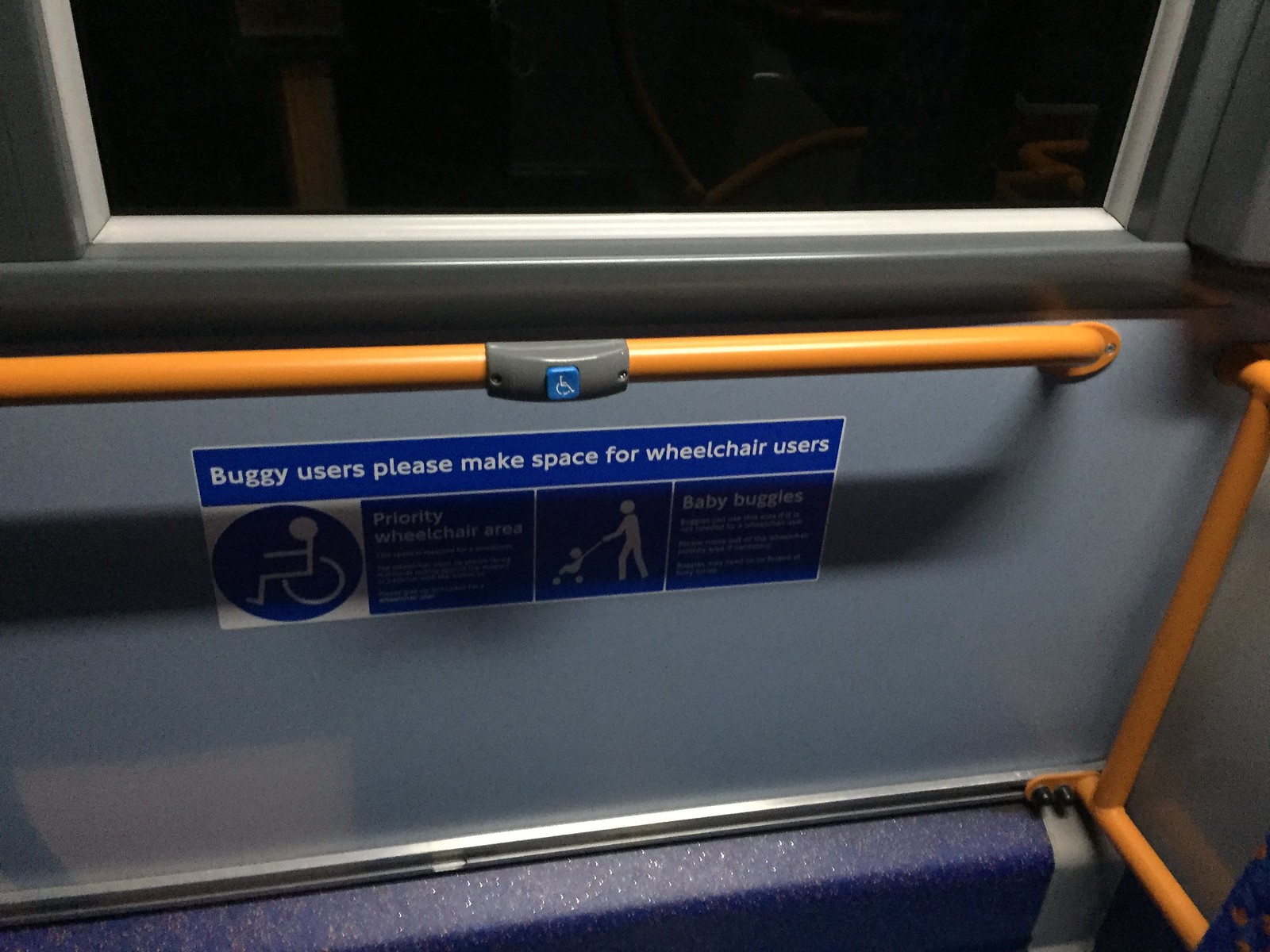This wide rectangular image captures the interior side of a train car or public transportation vehicle. At the top, there is a window bordered by white and gray metal, although it's impossible to glimpse anything outside as the window appears black. The dominant color scheme inside is grayish blue walls accented with bright yellow-orange poles. One pole runs horizontally across the scene, while another extends vertically on the right side. Affixed in the middle of the horizontal pole, there is a gray fixture with a blue square button displaying a white wheelchair symbol. Directly beneath this is a long blue sticker featuring stick figures and a message that reads, "Buggy users please make space for wheelchair users." The sticker also includes small text that is too small to read, with part of the sign showing a figure pushing a buggy with a child. The floor appears to be blue, and there is a window above the horizontal pole, underlining the utilitarian yet accommodating design of the public transportation space.